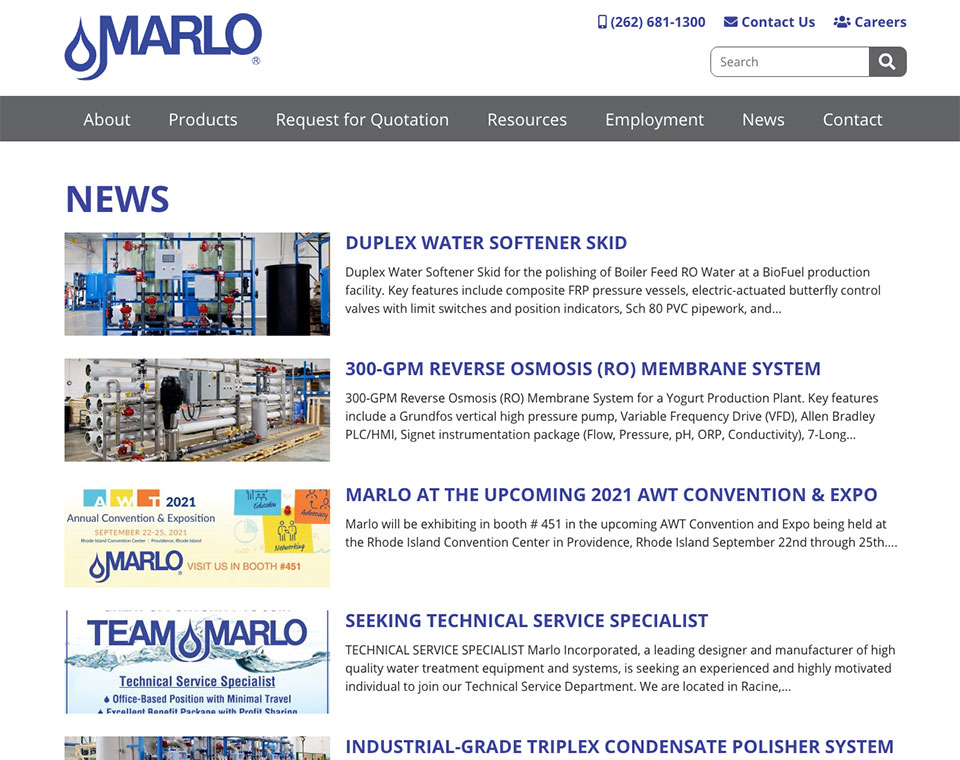The home screen of Marlowe’s website is depicted. In the top left corner, a blue icon represents the brand logo. Adjacent to the right, contact information, including a phone number, a "Contact Us" link, and a "Careers" link, is displayed. A search bar outlined in gray, featuring a gray magnifying glass icon, is located on the right side of the screen.

A horizontal gray banner runs across the top of the page, featuring the primary navigation options in white text: "About," "Products," "Requests for Quotation," "Resources," "Employment," and "News." These categories are clearly delineated to guide user navigation.

Below the banner, the word "NEWS" is prominently displayed in large, uppercase blue text. This section highlights several stories, each accompanied by a rectangular splash image. The headlines are also in the same blue color as the logo and the “NEWS” banner:

1. "Duplex Water Softener Skid"
2. "300 GPM Reverse Osmosis (RO) Membrane System"
3. "Marlowe at the Upcoming 2021 AWT Convention & Expo"
4. "Seeking Technical Service Specialist"
5. "Industrial Grade Triplex Condensate Polisher System"

Each headline is followed by a brief introductory sentence or two, giving an overview of the respective stories. The text provides an engaging preview, inviting readers to explore further details on each topic.